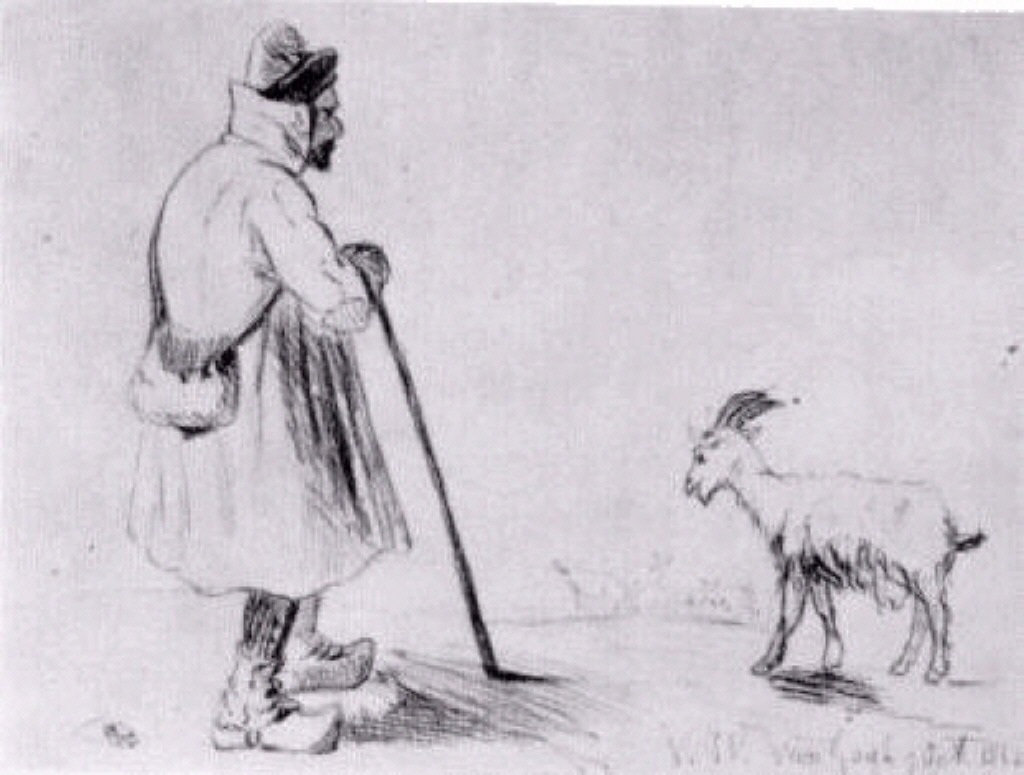"This detailed black and white pencil drawing, possibly on heavy stock paper or canvas, depicts a man standing in profile on the left side and a small white goat on the right. The man, who has a mustache and beard, is adorned with a unique cone-shaped gray hat and a long trench coat with an upturned collar that partially covers his face. He is holding a long black cane in his right hand and wearing distinctive upturned-toe boots. Across his body, he has a crossbody bag with its main compartment resting on his back. The goat beside him has two black horns and is standing amidst strands of grass, adding texture to the predominantly white background with various gray lines."